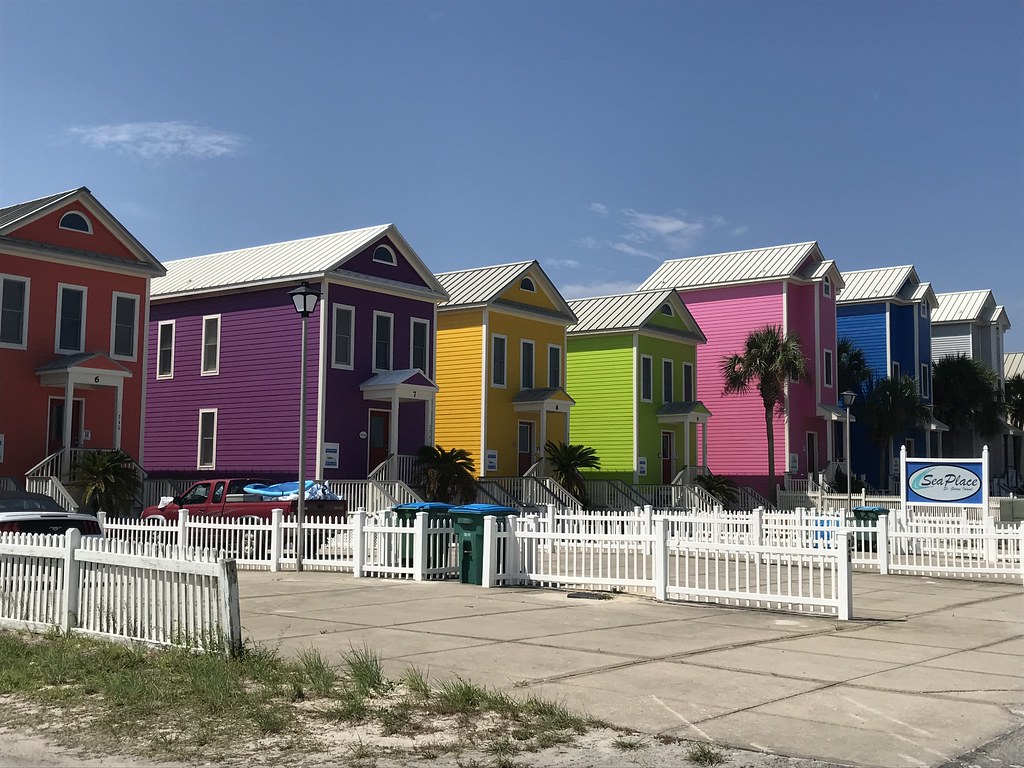The image captures a vibrant beachside community known as Sea Place. The foreground prominently features a row of colorful, narrow, two-story beach cottages lined with white trim. Starting from the left, the houses are painted in vivid shades of red, purple, gold, and lime green. Each house has a pristine white roof, yard lanterns, and palm trees outside. Moving further right, additional three-story homes appear in pink, blue, and gray, maintaining the charming color scheme with white trims.

A blue oval sign with white lettering, reading "Sea Place," is displayed prominently, confirming the name of this picturesque area. The houses front a totally concrete area that includes garbage pails and a parked truck, nestled between the homes and a white picket fence. Beyond the fence, sea grass grows, hinting at the vicinity of the beach. The streets are lined with more identical narrow homes, all meticulously maintained.

The sky above is a clear blue, dotted with puffy, scattered clouds, adding to the serene atmosphere of this lively beach community. Vehicles are visible in some of the driveways, completing the idyllic scene of Sea Place.